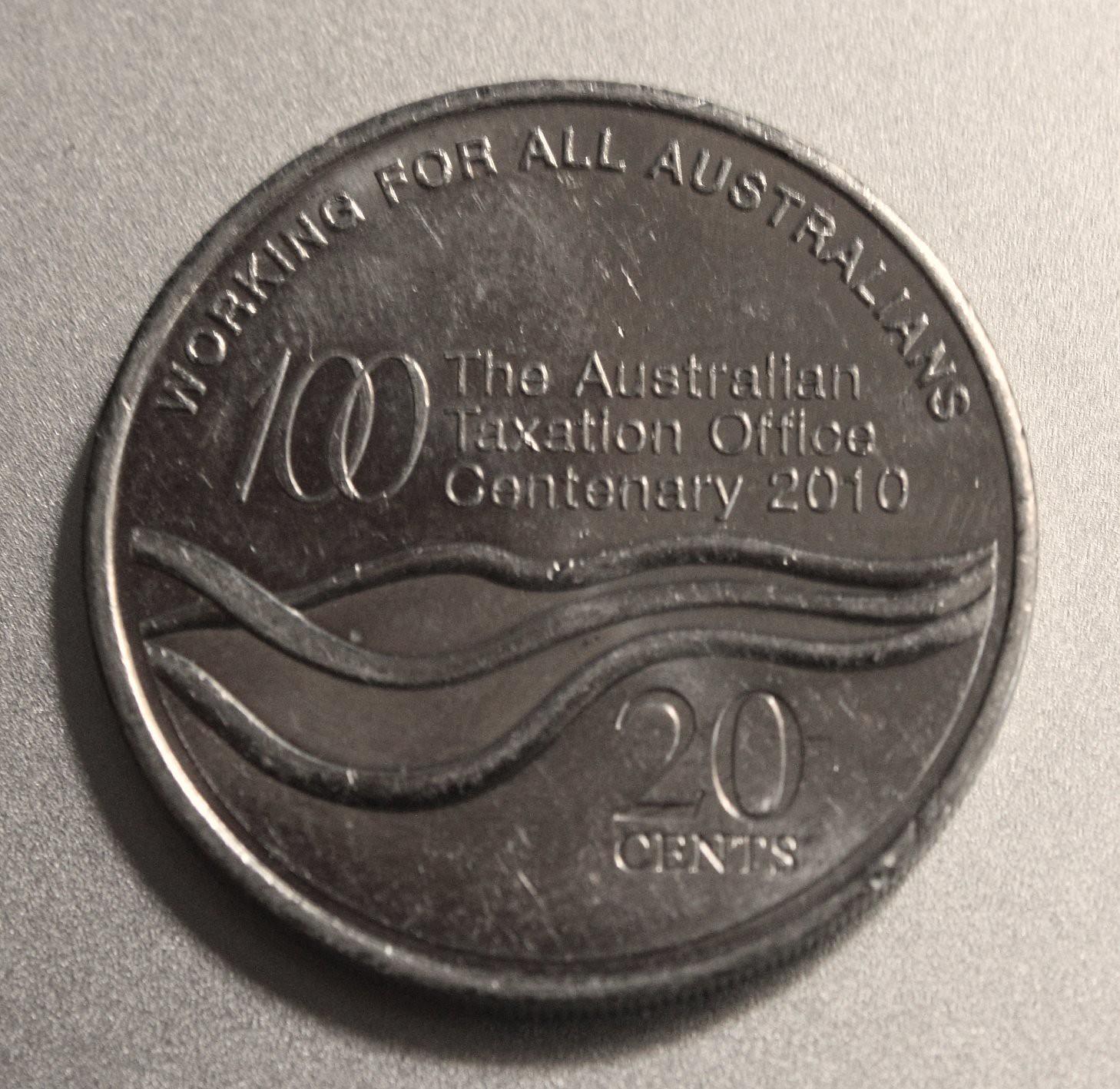The photograph captures a round, silver-colored coin resting on a grey patterned background. The coin's surface shows signs of wear, with visible scratches and blemishes. Surrounding the coin is an elevated, engraved border. The upper part of the coin displays the text "WORKING FOR ALL AUSTRALIANS" in all caps. Below this slogan, the coin commemorates the Australian Taxation Office with the inscription, "100, THE AUSTRALIAN TAXATION OFFICE, CENTENARY 2010," where the zeros are interlocked. The center of the coin features three wavy lines that converge from left to right. Beneath these lines, the denomination is marked as "20 cents," with the number "20" being indented, contrasting with the extruded text above. The overall patina and texture of the coin suggest it is not new, adding a historical context to this commemorative piece.